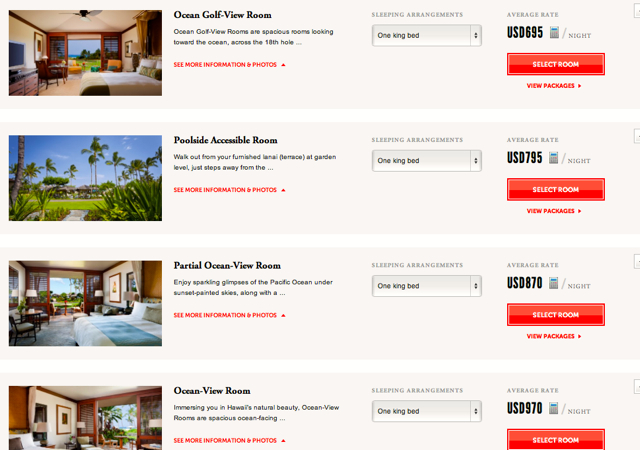The screen displays four room types at a tropical resort, each at different price points, arranged in ascending order from the cheapest at the top to the most expensive at the bottom. The first option, priced at $695 USD, is an Ocean Gulf View Room. This room features large screen doors that open onto a lush green golf course. Inside, there is a spacious king-size bed with a TV positioned at the foot of the bed, several armchairs, and a ceiling fan. 

The second option is a Poolside Accessible Room, providing direct views of the resort’s pool and surrounding palm trees. 

The third option is a Partial Ocean View Room, offering a glimpse of the ocean.

The fourth and final option, priced at $970 USD, is an Ocean View Room, providing an unobstructed and expansive view of the ocean. Each room is depicted with detailed images showcasing their unique features and offerings.